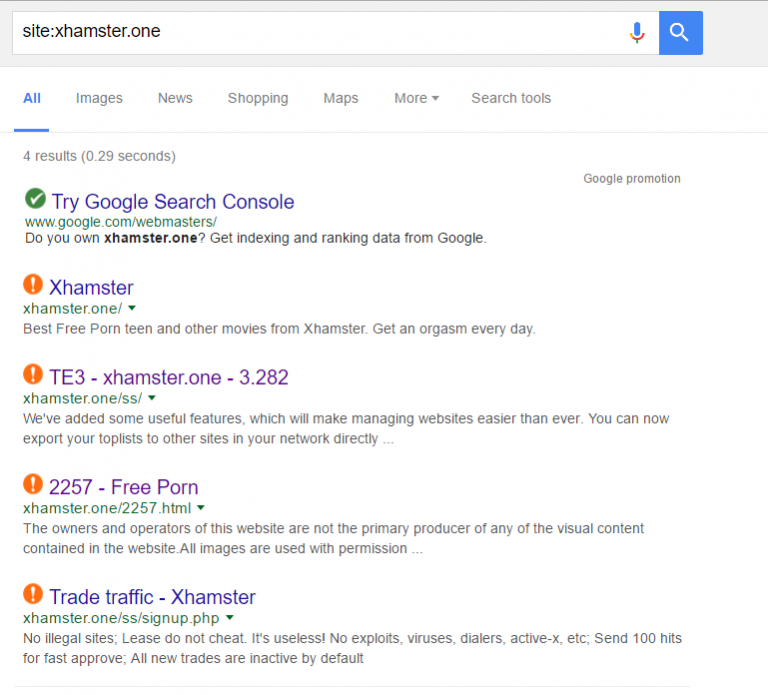Screenshot of Google search results for "site:xhamster.one"

In the search bar at the top, "site:xhamster.one" is entered. To the right of the search bar, there is a microphone and a magnifying glass icon, the latter serving as the search button. Below the search bar, there are navigation options labeled "All," "Images," "News," "Shopping," "Maps," and "More" with an accompanying drop-down arrow, followed by "Search tools."

The search results indicate there are four results found in 0.29 seconds. The first result recommends using the Google Search Console, with a link to "Google Promotion" (www.google.com/webmasters), asking, "Do you own xhamster.one? Get indexing and ranking data from Google."

The second result displays an orange circle with an exclamation point and a link to "xhamster.one" with a description stating, "Best free porn, best free teen porn, and other movies from xhamster. Get an orgasm every day."

The third result also shows an orange circle with an exclamation point with the title "TE3-xhamster.one-3.282" and a link to "xhamster.one/SS." The description reads, "I want to take a hit. We've added some useful features, which will make managing websites even easier than ever. You can now export your top list to other sites in your network directly..."

The screenshot is cropped, and additional search results are partially visible at the bottom.